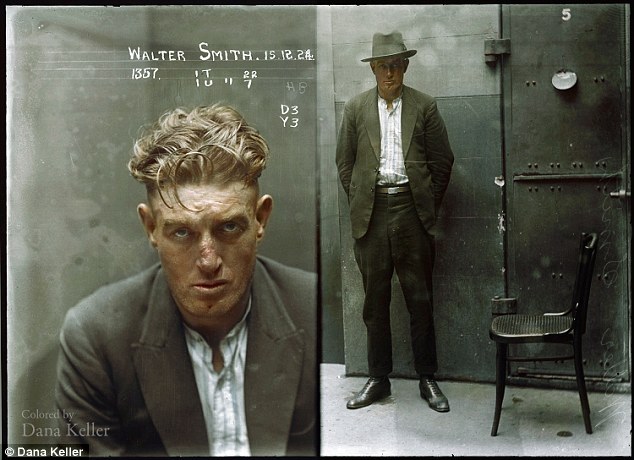This image is a meticulously colorized mug shot of a man named Walter Smith. The photograph, colored by Dana Keller, is likely an originally black-and-white picture that has been enhanced to offer more vivid details. The main portrait on the left displays Walter Smith, who appears disheveled with short, dirty blonde hair and a visibly scuffed face. He is attired in a dark gray suit jacket over a striped powder blue and white shirt, though he lacks a tie. The handwritten text above the mug shot includes various identifiers such as the date December 15, 2024, and perhaps prisoner identifiers like 5th 1357 IU 22 d3 y3.

Adjacent to this, the image on the right captures the same man standing, now with a black hat, black leather shoes, and a pair of pants, beside a black chair. The background reveals a stark setting with a wall featuring the number five, light gray paint on the upper section, and dark gray paint below. A door constructed of metal, presumably leading out of his holding area or prison cell, is also visible. This meticulously detailed image offers a blend of historical and forensic interest, portraying both the individual and his environment in striking color and detail.